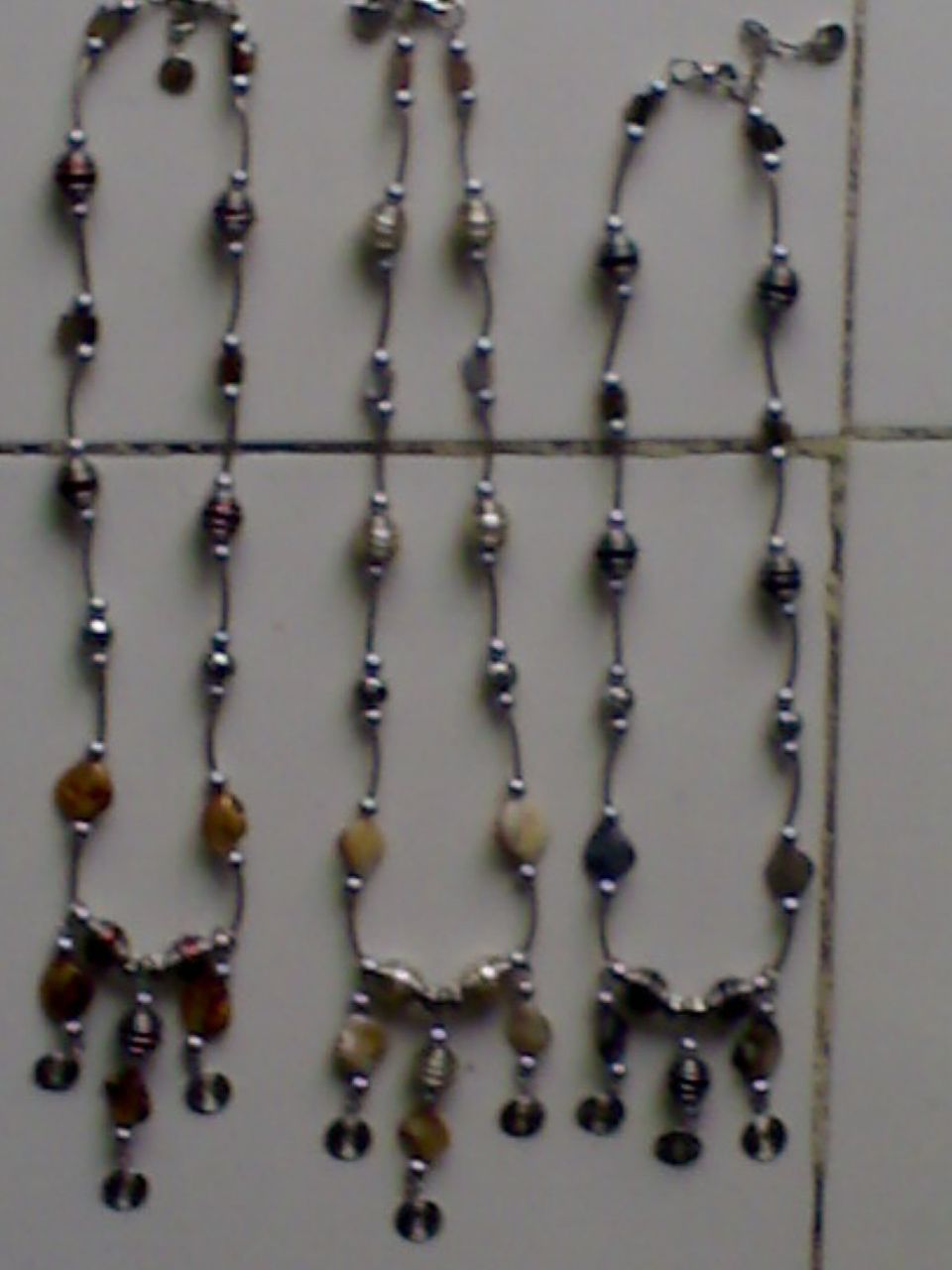The image shows three bead necklaces arranged side by side on a white tiled surface, which could be a wall or a floor, with black and yellow grout visible between the tiles. Each necklace, featuring small round beads connected by strings, hangs against the white tiles in a somewhat blurry photo. The necklace on the left has red beads, the middle one has yellow beads, and the one on the right has dark brown beads. Each necklace culminates in a similar pendant design: three hanging beads each extending into circular discs, resembling musical notes with varying colored components. The necklaces exhibit slight variations in their pendant lengths and colors but share a cohesive overall design.